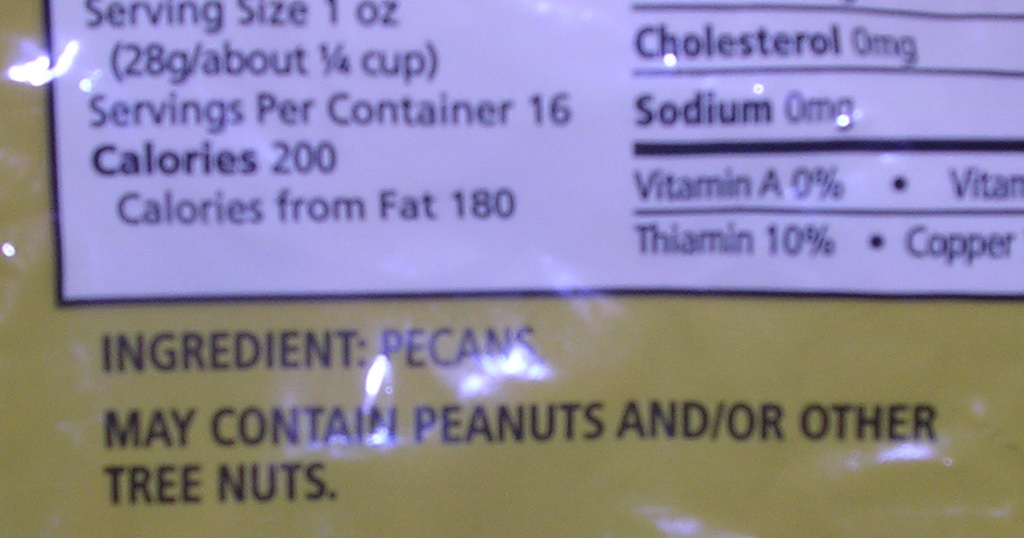The image depicts the bottom portion of a Nutrition Facts label on the back of a glossy, yellow snack bag with a prominent glare from a light source at the top left corner. The label, set on a white background with black text, lists the nutritional information for a serving size of one ounce (28 grams), approximately a quarter cup, with 16 servings per container. Each serving contains 200 calories, with 180 calories from fat, zero milligrams of cholesterol, zero milligrams of sodium, and provides 0% of the daily value for Vitamin A and 10% for thiamin. Below the nutritional information, in a brown rectangle with black text, are the ingredients listed as pecans. It also mentions that the product may contain peanuts and/or other tree nuts. The detailed information and reflections on the bag suggest a highly reflective surface.